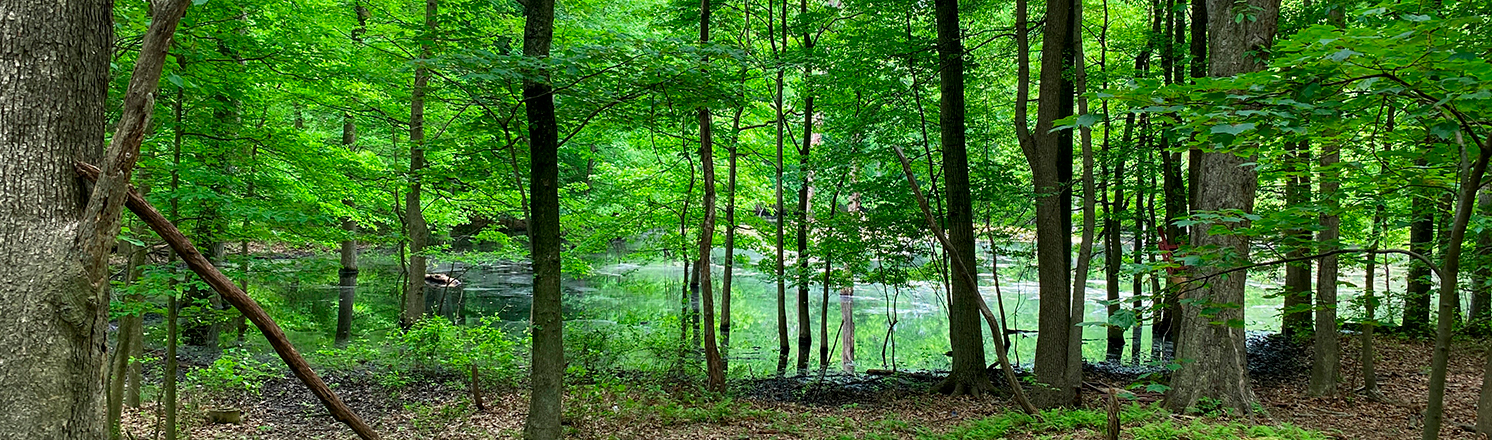The panoramic image captures a dense forest scene during the daytime, characterized by a mix of vibrant green foliage and brown, crunchy leaves on the forest floor. The tree trunks vary in thickness, with some appearing robust and ancient while others are thinner and wiry, indicating a diverse age range among the trees. In the foreground, the ground is covered with dead leaves and dirt, particularly noticeable on the right and left sides. Sprinkled among the leaves are twigs and branches, adding to the forest's natural clutter.

A prominent feature is a still body of water, possibly a pond or small lake, located in the center of the image. This water body reflects the surrounding trees and sky, giving it a glassy, almost whitish appearance in places where the sunlight hits. The reflection in the water enhances the depth and tranquility of the scene. In contrast to the predominantly brown forest floor, thick green moss adds texture to the pond, accentuating the forest's lushness. The canopy above is filled with myriad green leaves that filter the sunlight, creating a vibrant, tranquil atmosphere. The sunlight particularly highlights the center area, making the green leaves appear even more vivid and lively.